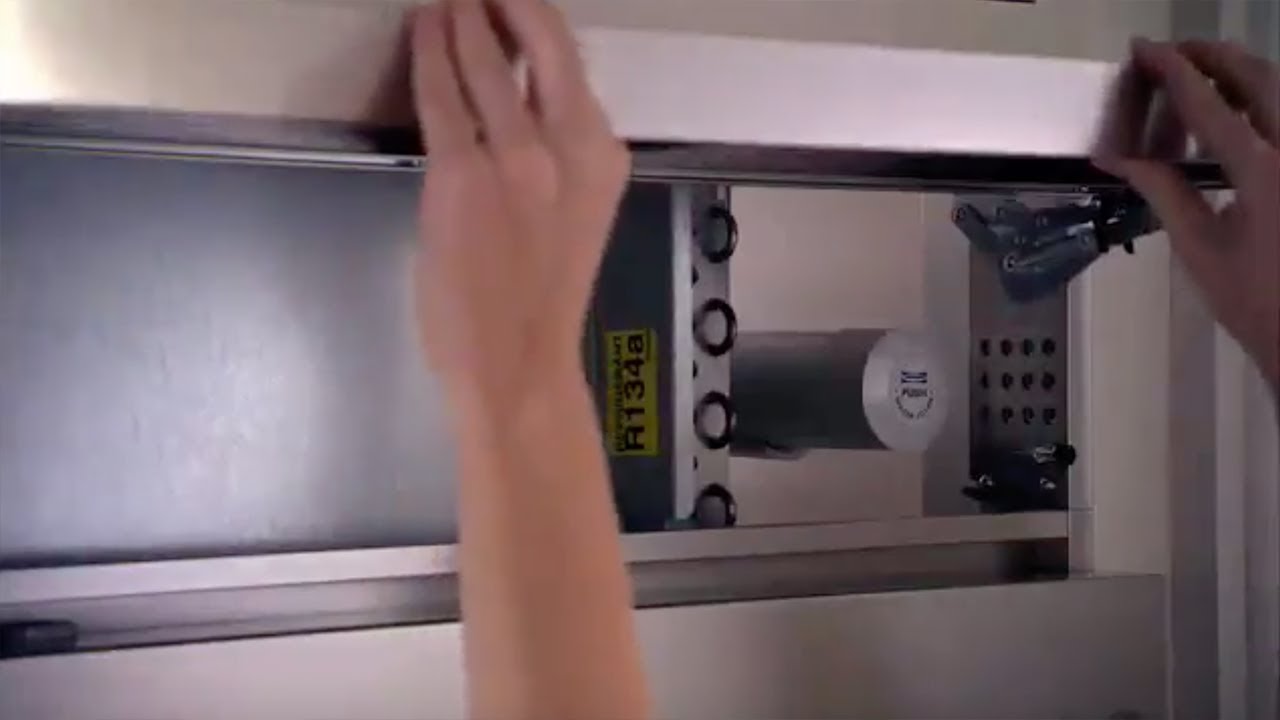A Caucasian individual is working on a rectangular, silver mechanical box mounted on a white wall. The box appears to be some sort of industrial equipment or machine. Its steel sliding door has been opened and slid to the left, revealing the interior. Inside, there's a prominent gray cylindrical component with some indecipherable writing on its front. The cylinder is flanked by small walls on both sides. The left wall features a long, flat gray panel, while the right wall has a metal plate with perforated holes. There is a yellow label with the code "R1348" on the front. The top and bottom sections of the machine are bordered with silver paneling. Two white hands are interacting with the mechanism: the central hand appears to be gripping the edge of the sliding door, while the right-hand side seems to be holding or placing an object near the equipment.